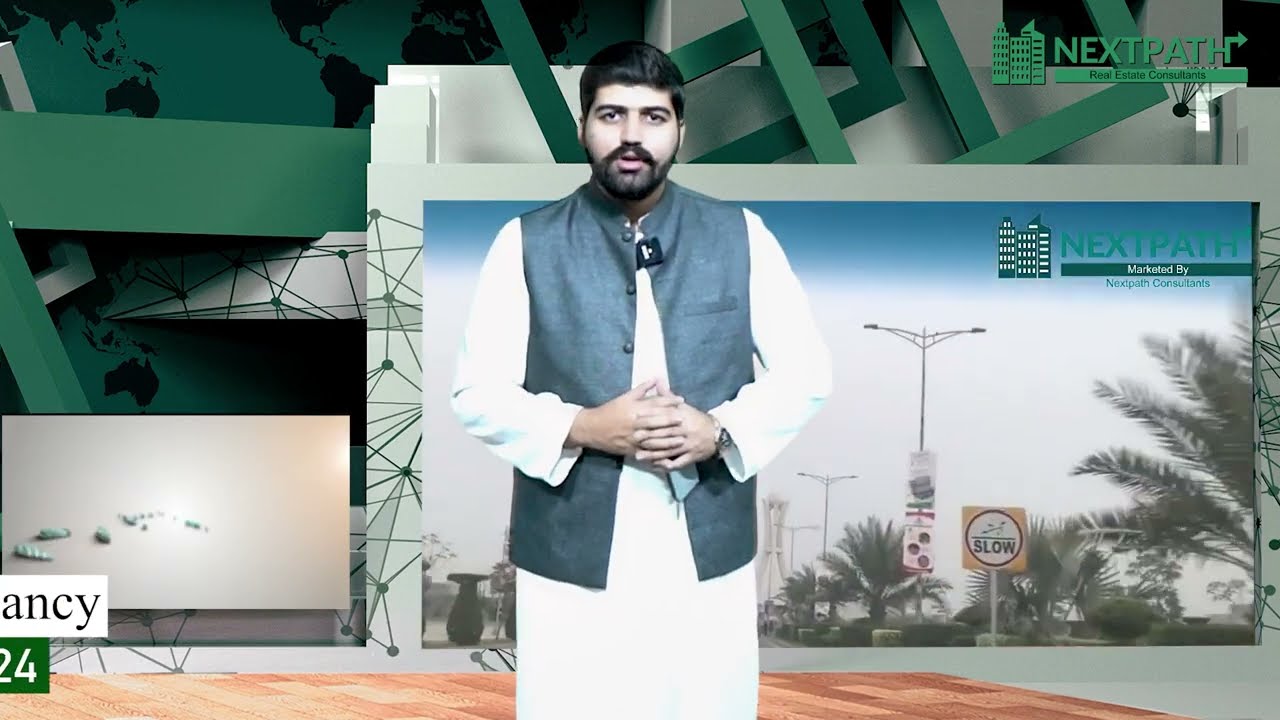The image captures a Middle Eastern man standing as if he is reporting on television, possibly for a news segment or a web production. He has a neatly combed back head of dark black hair and a full black beard, accentuated by thick black eyebrows. His hands are clasped together in front of him, displaying a watch on his right wrist. He is dressed in a traditional white robe, over which he wears a gray vest.

Behind him, the backdrop appears to be a digitally created or green-screened image featuring various elements. Dominating the upper right corner are the words NextPath Real Estate Consultants in green lettering, accompanied by an illustration of three skyscrapers. Below this, there is a line of text indicating "NextPath marketed by NextPath Consultants," though some finer details are indistinguishable.

Further details in the background include an image of a street lined with palm trees and streetlights. A sign bearing a yellow square with a red circle reading “slow” is also visible. Geometric green designs with an architectural theme and black silhouettes of world maps, including regions like Africa, Australia, and the United States, blend into the scene, adding depth and complexity to the backdrop. Additionally, the bottom left corner of the image showcases the fragmented letters "A-N-C-Y" in black text on a white background, with the number 24 in white text on a green background beneath it.

This comprehensive description highlights the intersection of traditional attire with a modern, possibly virtual, backdrop, suggesting the man may be involved in a real estate presentation or a news broadcast for NextPath Real Estate Consultants.